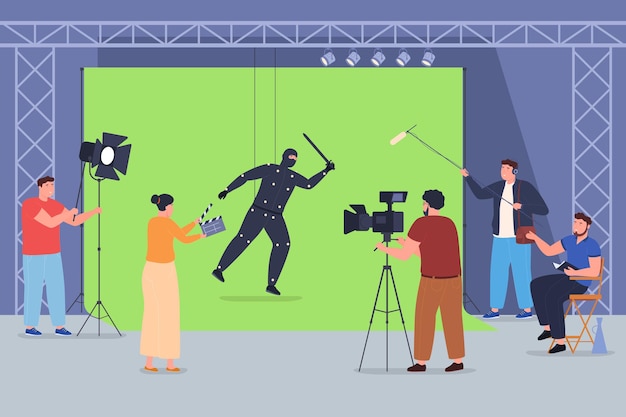The scene is an animated movie set, intricately drawn in a digital style, capturing a dynamic and meticulous depiction of a film production. At the center of the image is a male actor, clad in an entirely black suit that encompasses black shoes, pants, shirt, gloves, mask, and headpiece. His face is mostly obscured, revealing only his eyes and a bit of his nose through the suit. Small white motion sensors are affixed to various points on his outfit. The actor is suspended in mid-air, supported by two wires, and is positioned in front of a vivid green screen.

The bustling set is populated by five crew members, each meticulously engaged in their roles. One holds a boom microphone above the actor, capturing audio. Another, a bearded man dressed in all brown with dark shoes, stands behind a professional video camera mounted on a tripod, diligently filming the scene. A woman, in an orange top and a lighter-colored skirt, holds a clapperboard, poised to mark the start of takes. Another crew member is responsible for handling the lights aimed at the actor, ensuring proper illumination. An array of lights is suspended from a metal apparatus, which frames the dark gray background, providing additional lighting for the scene.

The director, distinguishable by his seated position and megaphone, oversees the entire operation, orchestrating the various elements. The entire setup sits on a gray slate floor, further grounding the scene in a realistic setting, despite its animated depiction. The image beautifully encapsulates the coordination and effort involved in bringing cinematic visions to life.